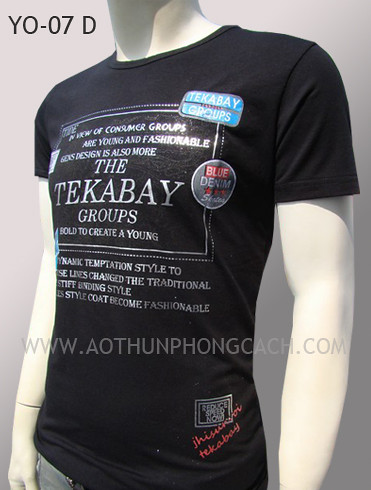The image depicts a white mannequin dressed in a black t-shirt and jeans. The black t-shirt features prominent white lettering across the chest that reads "The Teka Bay Groups." Below this, the text "Ayung and Fashionable" is visible, highlighting a modern and trendy design style. The text also mentions a shift from traditional stiff binding styles to more contemporary and fashionable codes. The URL "www.aothongcash.com" is inscribed in light gray letters across the t-shirt. The top-left corner displays "Y07D" in black letters. The mannequin’s arms hang by its sides, and its stark white color contrasts sharply with the dark t-shirt.